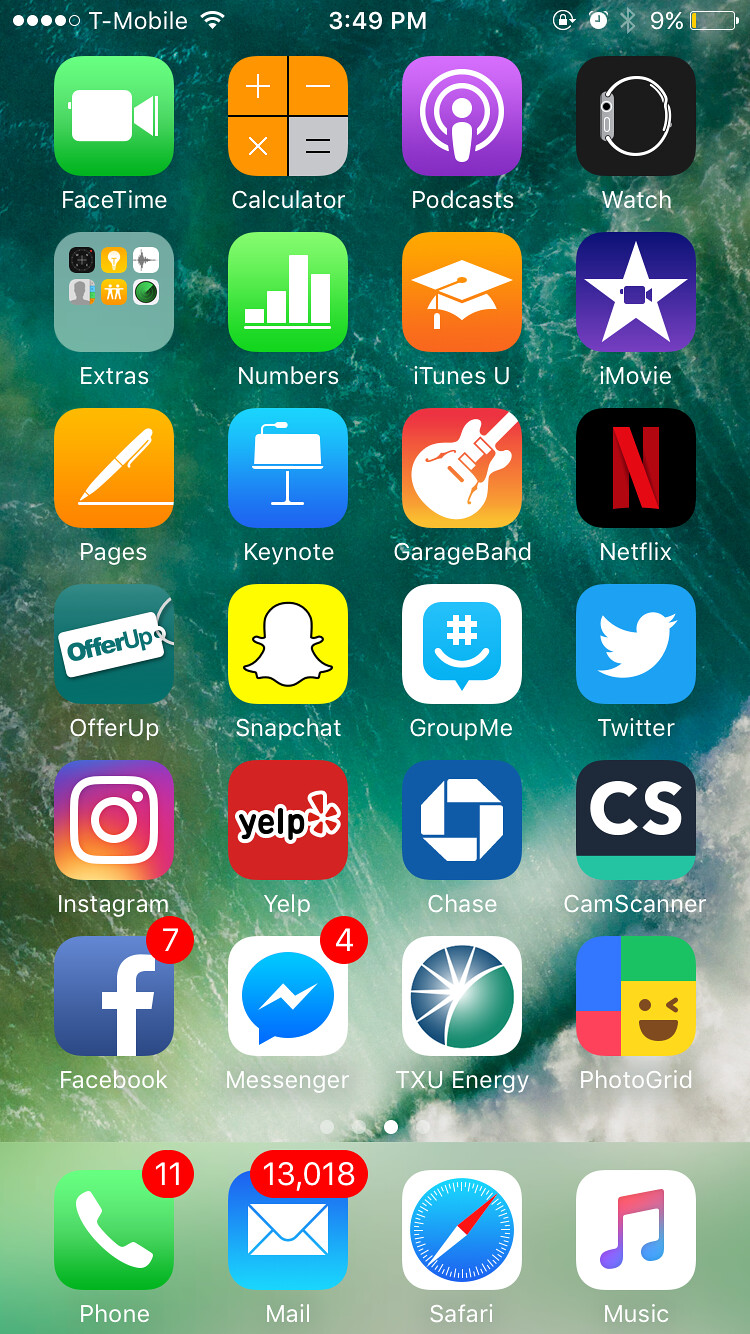This screenshot, captured from a cell phone, showcases a vibrant and busy home screen. At the top, the phone is connected to T-Mobile with an active Wi-Fi connection, displaying the time as 3:49 PM and indicating a critically low battery level at 9%, along with an active Bluetooth connection. The background image features a dark green marbled design, possibly depicting an ocean wave intermixed with white accents.

The home screen is densely packed with a variety of apps and icons. Featured prominently are the FaceTime app in green, a calculator, and a purple Podcasts button. A black button for the Watch app is also present. Additionally, there's an "Extras" folder. Notable apps include Numbers, iTunes U, iMovie, Pages, Keynote, GarageBand, Netflix, OfferUp, Snapchat, GroupMe, Twitter, Instagram, Yelp, Chase, CamScanner, Facebook, Messenger, TXU Energy, and PhotoGrid. At the bottom of the screen, the frequently used icons for Phone, Mail, Safari, and Music are neatly aligned.